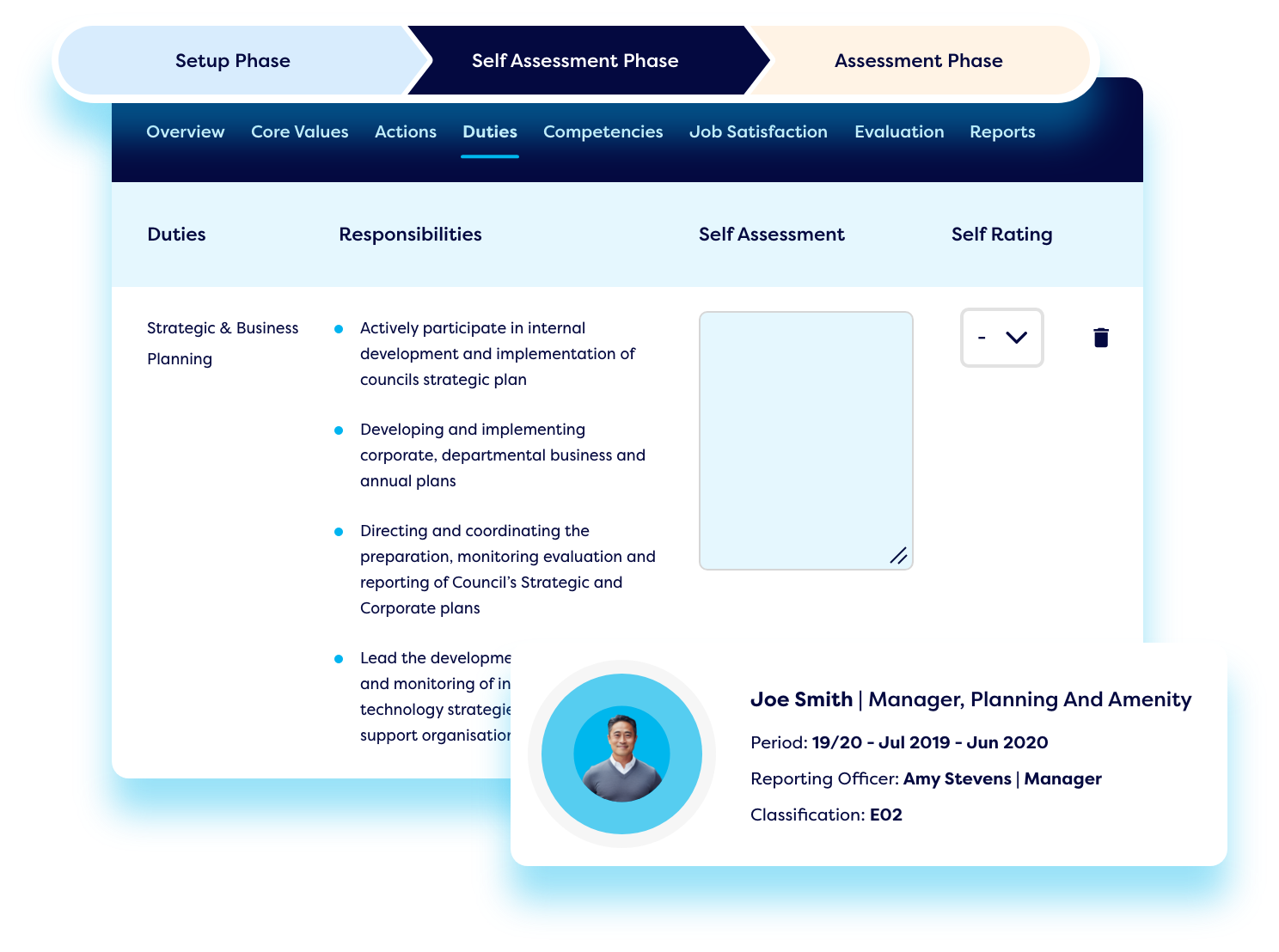**Caption:**

Joe Smith, the Manager of Planning and Amenities, is depicted in the image taken during the setup phase of the self-assessment process for the period of July 2019 through June 2020 (Period 19-20). In the evaluation process supervised by Amy Stevens, the Reporting Officer with a classification of E02, Joe is dressed in a gray sweater with a white collar, complementing his short black hair. The process entails phases including Self-Assessment and Assessment, focusing on various aspects such as an overview of core values, actions, duties, competencies, and job satisfaction. Evaluation reports are crucial, where duties and responsibilities, as well as self-assessment ratings, are meticulously examined.